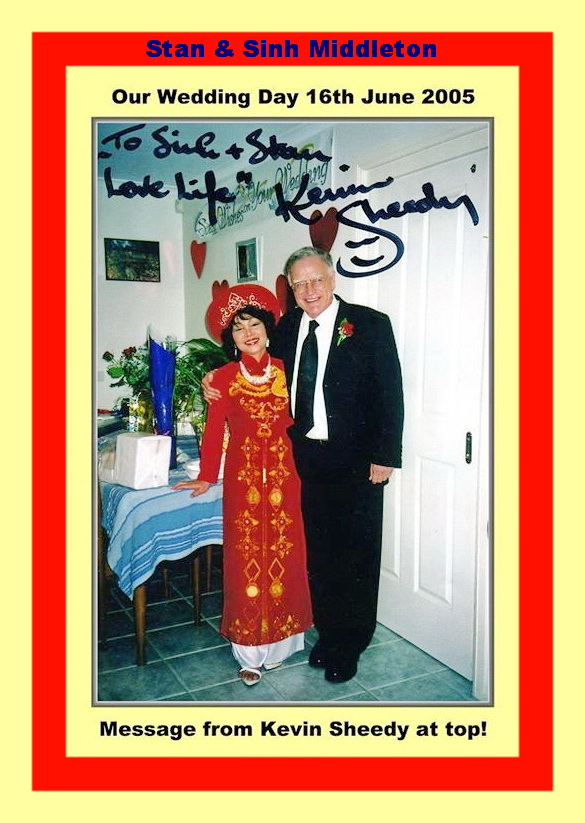This image, framed by a tan border followed by a thin red one, showcases "Stan and Sin Middleton" in elegant blue font. Within the inner tan border, it reads “Our Wedding Day, 16th June 2005.” Handwritten at the top in black sharpie is “To Sue and Stan, love life,” signed by Kevin Sheedy. The photograph features a joyful couple, presumably Stan and Sin Middleton, standing in what appears to be their home. The woman, on the left, is dressed in a fancy red and gold dress with a white bottom, accessorized with a matching red hat, red lipstick, and black curly hair. The man, on her right, has his arm around her, dressed sharply in a black tuxedo with a white shirt, black tie, and a red flower pinned to his lapel. They are both smiling warmly. Behind them is a table with a blue-striped tablecloth set against a backdrop of flowers, gifts, framed pictures, a white door, and a blue-tiled floor, capturing a moment of happiness and celebration on their wedding day.